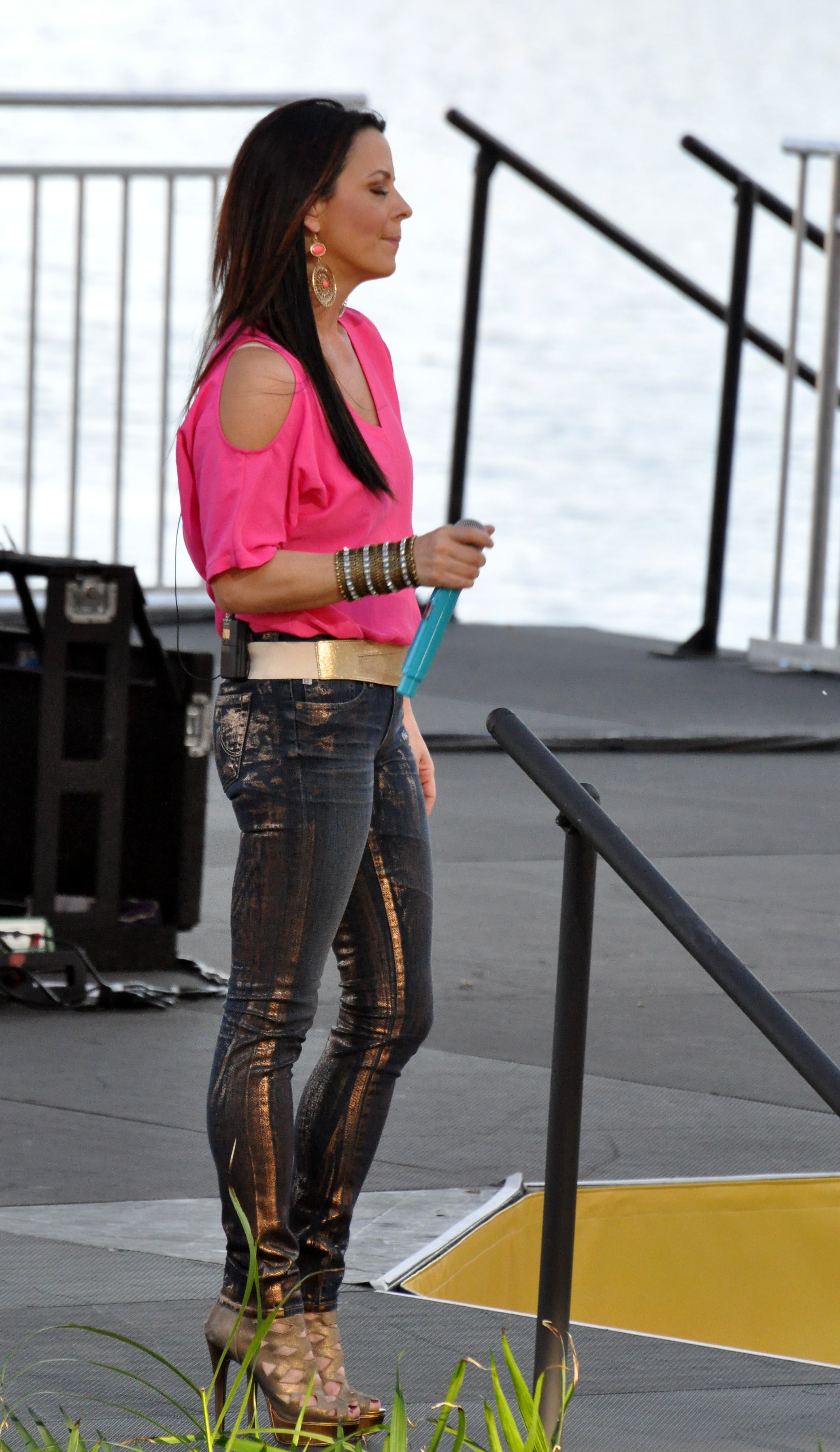A performer stands on a stage, facing the right side of the image. She is dressed in skin-tight, black leather or plastic-like pants, accented by a gold streak down the left side, and a short-sleeved pink top with circular cutouts revealing her shoulders. A gold belt cinches her waist, while her feet are adorned with high stiletto heels in a gold or brown hue. Her right hand, which is bent at the elbow, holds a blue microphone, complemented by a thick wristband decked with four rows of sparkling jewels. Her long black hair cascades over her shoulders, framing pink earrings. The background features a blurry ocean view, with stairs and a metal fence visible, alongside sound equipment on the left, indicating she is likely a singer either about to perform or having just finished a song.